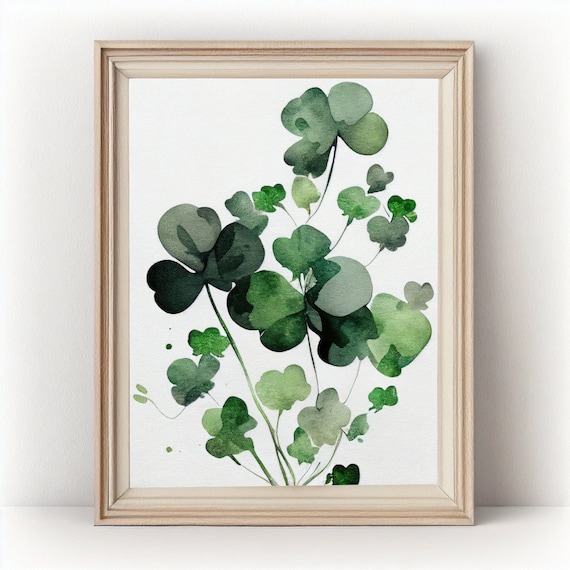The product photograph showcases a rectangular piece of artwork set in a light brown wooden frame against a solid white surface and background, typical of commercial listings like online shops, catalogs, or web pages. The artwork itself, likely a watercolor, features multiple green clovers on thin green stems growing from the bottom of the frame. The clovers, varying in shades from light green to dark green with some approaching grayish-black, mostly have three to four leaves. The painting, displaying an impressionistic quality with splotches and splashes of color, is set on white paper. The simplicity of the natural wood frame complements the minimalist aesthetic of the image, making it suitable for various commercial purposes.